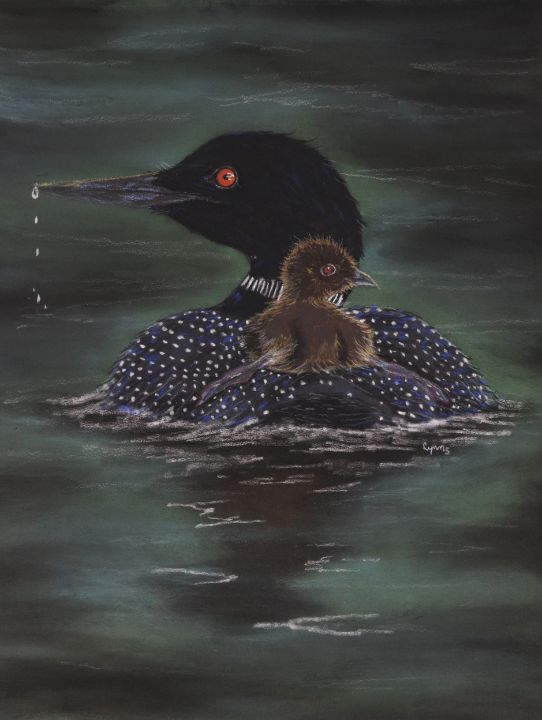This color painting, in portrait orientation, presents an incredibly realistic depiction of a waterfowl and its young. The scene centers on a large aquatic bird, likely a loon, gliding across a blackish-green pond with hints of white ripples trailing behind. The adult bird is painted with meticulous detail: its black head has a striking red eye and a long black beak from which water droplets drip. A distinctive white dashed line rings its neck, and its dark gray body is speckled with a pattern of white dots. The bird faces the left side of the image, providing a side profile view of its head.

Perched on the adult's back is a fuzzy, dark brown juvenile, sparsely decorated with black specks and featuring a subtler red eye. The baby bird, contrasting its parent, looks to the right. Both birds float serenely in the water, with the adult partially submerged, showcasing the seamless blend of their forms with the aquatic environment. This meticulous depiction captures the intimate and tender moment between the adult waterfowl and its offspring.